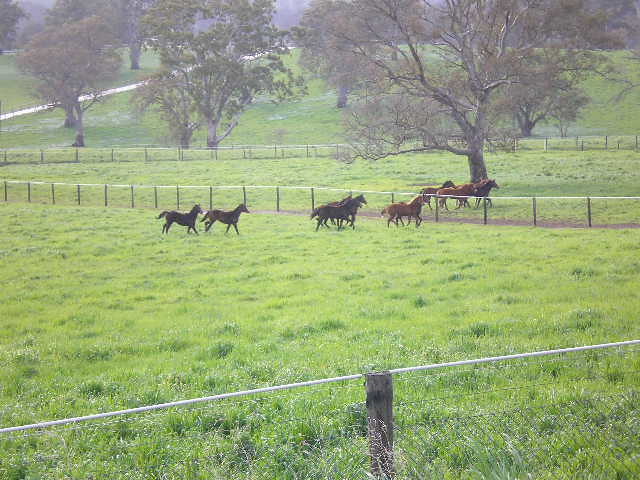The photograph captures a misty outdoor scene centered in a large, grassy field. The lush green grass, ankle-length and fluffy, spreads throughout the image, giving it a serene, foggy morning or cloudy day ambiance. The field is divided by multiple metal fences with sturdy wooden posts, one prominent in the foreground. Scattered across the field, groups of dark brown and black horses, predominantly adults, are seen running and standing, creating a lively yet tranquil atmosphere. Most horses, a mix of five in the nearest section and three farther back, are positioned centrally in the photograph, facing right. The background features a rolling landscape with green hills adorned by scattered trees and a visible road to the left. These trees, primarily bare with dormant branches, add to the atmospheric, slightly obscured view. The overall grainy texture of the image softens the finer details, enhancing the dreamy, idyllic quality of this pastoral scene.